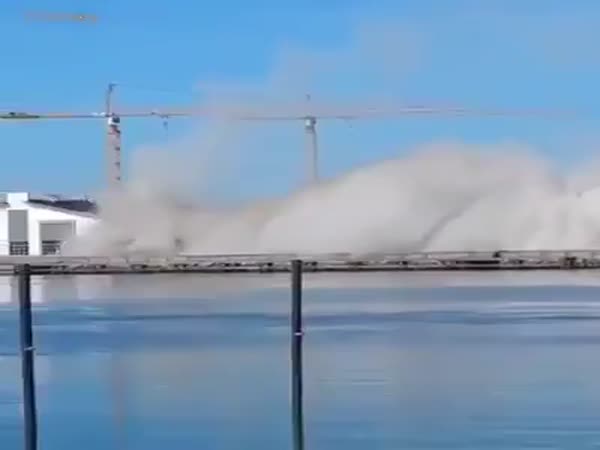The image depicts a scene with a bright blue sky devoid of clouds. Prominently in the foreground is a body of water, likely part of an ocean or bay, partially enclosed by what appears to be a glass wall. There are two vertical black poles emerging from this area, their purpose unclear but they could be part of a railing or pier structure. The focal point is a large, cloud-like mist rising from the water, suggesting recent activity—perhaps a boat moving swiftly past.

In the background on the left, there's a white building, potentially a part of a marina. To the right of this structure, two large crane-like forms or control towers stand, identifiable by their arms extending outward. These tower over a ground layer shrouded in a thick, gray smoke or dust, obscuring other possible details. The entire landscape behind the mist looks hazy, blending into the bright sky and masking further specifics.